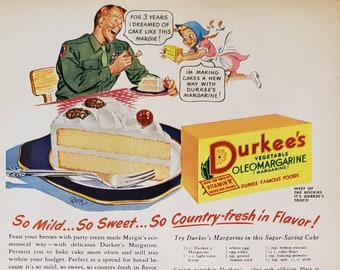This vintage advertisement for Dierke's margarine features an off-white to light beige background in a nearly square format. Dominating the top left is a cartoon scene: a man in a military uniform beams with delight as he sits at a table adorned with a red and white checkered cloth, enjoying a slice of cake. A dialogue bubble above him reads, "For three years I dreamed of cake like this." Beside him runs a little girl, dressed in a pink dress, white apron, and blue bonnet, holding a yellow box of margarine. Her dialogue bubble proudly declares, "I'm making cakes a new way with Dierke's margarine."

At the center of the image is an illustration of a piece of white cake, while to the right is a yellow box of Dierke's margarine. The box features the brand name in red letters, with a flower dotting the "i" in "Dierke's," and below it in dark green or black, it reads "vegetable oleo margarine." Further down, the text "So mild, so sweet, so country fresh in flavor" appears in wavy red lettering. At the bottom of the advertisement, a recipe and additional text are displayed, rounding out the nostalgic and detailed promotional piece.